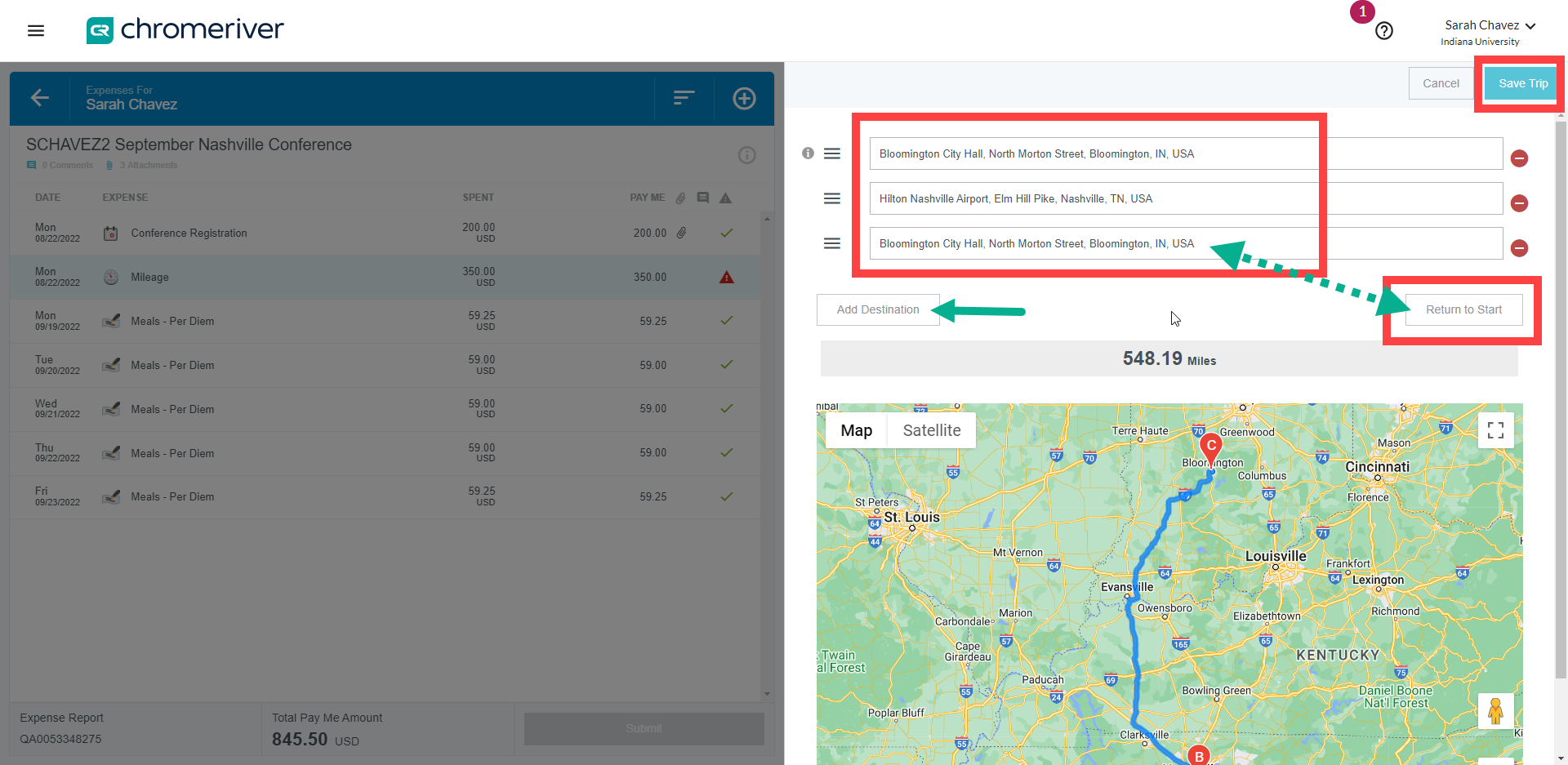This series of screenshots appears to be from either a mobile device or a website, featuring what looks to be the interface of an expense reporting tool named Chrome River. 

On the left side of the image, the background is grayed out, suggesting a pop-up overlay on the website. The top-left corner features three horizontal black bars against a white background, commonly indicating a menu. To the right of the bars is a green square with the white letters "CR," followed by the text "Chrome River" in black lowercase letters.

Underneath, the grayed-out section displays a green bar at the top with "Sarah Chavez" in white on the left, and on the right, a white plus sign inside a circle adjacent to three horizontal lines. Below this bar, the text "Chavez 2, September Nashville Conference" is visible in black. An overlay displaying a mileage and expense report appears on the left-hand side, with the text "Expense Report" at the bottom and a summary in the center stating "Total Pay Me Amount: $845.50 USD."

On the right-hand side of the image, there is an open map window. The map contains a red dot with a white "1" at the upper right corner and a question mark inside an information circle in black. Adjacent to this, the name "Sarah Chavez" appears in gray, followed by "Indiana University" with a down arrow. The top-right corner features a large blue rectangular button outlined in thick red that says "Save Trip" in white, while next to it is a white button labeled "Cancel."

On the left-hand side within another red-outlined area are three filled fields: "Bloomington City Hall," "Hilton Nashville Airport," and "Bloomington City Hall" again. A green arrow points within this red outline to a smaller red square on the bottom right labeled "Return to Start." Additionally, on the left, there is a white button that says "Add Description," also indicated by a green arrow.

Beneath these sections, a gray bar reads "548 miles" in black text. Below this bar is a green map section showing a route marked from Point B to Point C with a blue line in between, located between St. Louis and Louisville.